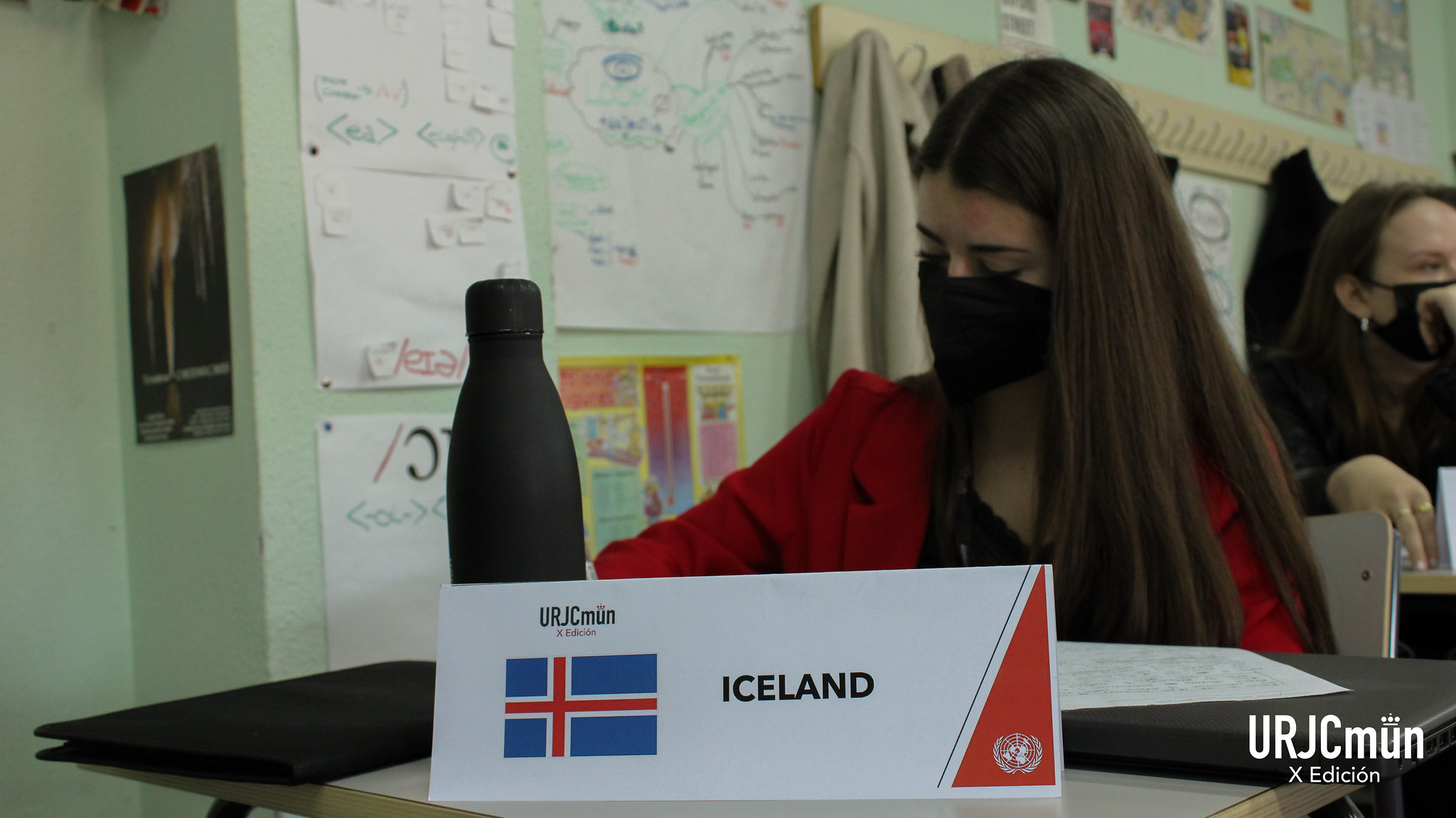The image depicts a young woman in a classroom setting, likely during the COVID-19 pandemic, given the black face mask covering her nose and mouth. She has long, straight dark hair and is wearing a red jacket over a black top. She is positioned slightly right of center in the photograph, sitting at a desk with her eyes looking down at a piece of paper, appearing to write. On her desk, there is a prominent sign labeled "Iceland" featuring a blue and red flag, along with some undecipherable writing and a red triangle symbol. A black water bottle stands to the left of the sign, and a black folder is visible nearby. Behind the main subject, pinned calendars and various papers adorn the green walls, and a coat is seen hanging. A second woman with dark hair, also wearing a black mask, is seated at a desk behind her. In the bottom right corner of the image, the letters "U R J C" followed by "M U N" and the smaller text "X edition" can be seen.